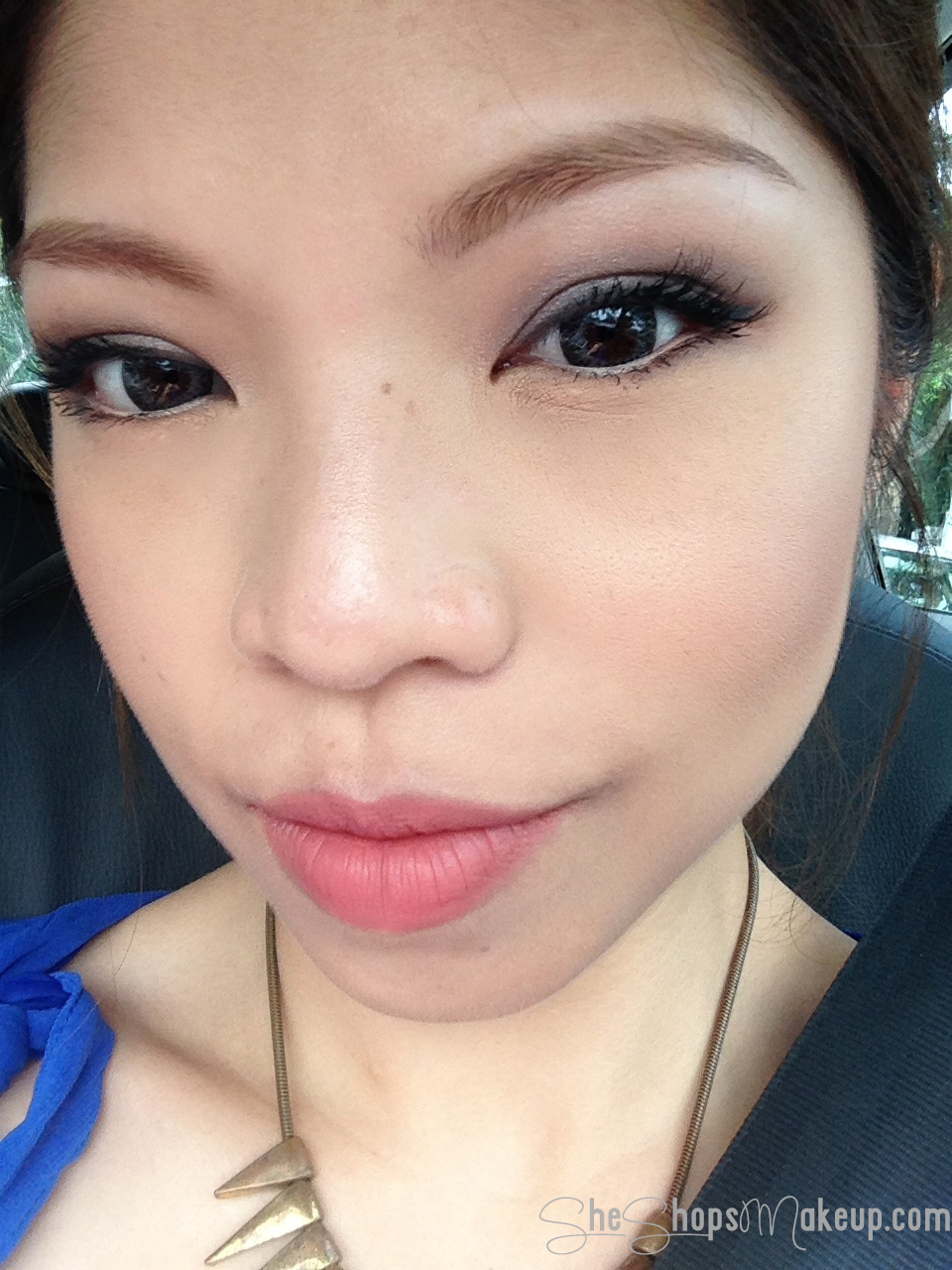The image is a close-up photo of an Asian woman with fair skin, captured from an angle that gives a slight fish-eye lens effect. Her black hair is pulled back, and she has dark brown, nearly black eyes accentuated with black eyeliner and blue-gray eyeshadow. Her eyebrows are also brown, and she's wearing pitch-colored lipstick. The woman is slightly smiling, enhancing her delicate features. She has a bronze-colored necklace adorned with triangular metal pieces resting against her neck. She is dressed in a light blue top, with fabric draped over her shoulder. Part of a seat belt is visible on the bottom right of the image, indicating she is seated inside a car. The background shows some greenery visible through the car window, adding a natural touch to the scene.